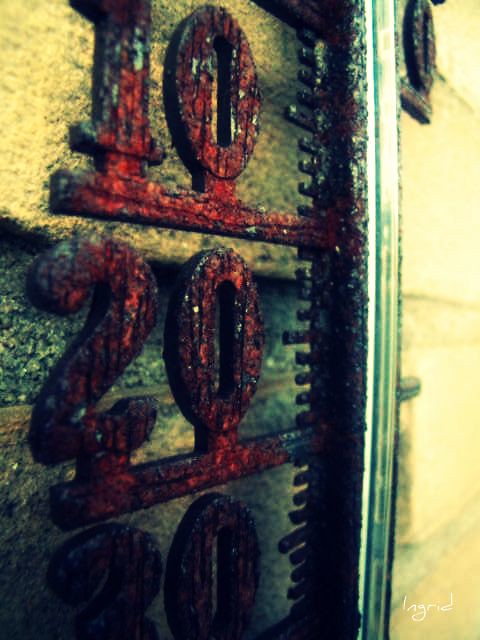The image depicts a rustic, antique measuring scale with a giant ruler-like appearance. The scale is marked with both centimetre and millimetre measurements, with the larger, prominent numbers displayed at intervals of 10 (10, 20, 30, etc.). These numbers are in a bold, oversized font. The structure appears to be made of wood, as indicated by the visible grain lines, though it also has spots of rust or mould, suggesting a degree of age and wear.

The scale's overall colour is a weathered, rustic red, complementing the sense of antiquity. The background of the image is dirty, featuring a creamy beige to yellowish hue with horizontal slats, adding to the old-world aesthetic. In the top right corner, there is a smaller number, possibly a zero, though its purpose is unclear in the context of the image. 

This measuring scale could be mounted on the side of a building or used for measuring height, given its large format and detailed gradations. The blend of iron and wooden elements, along with the backdrop, gives the scene a vintage, slightly neglected appearance.